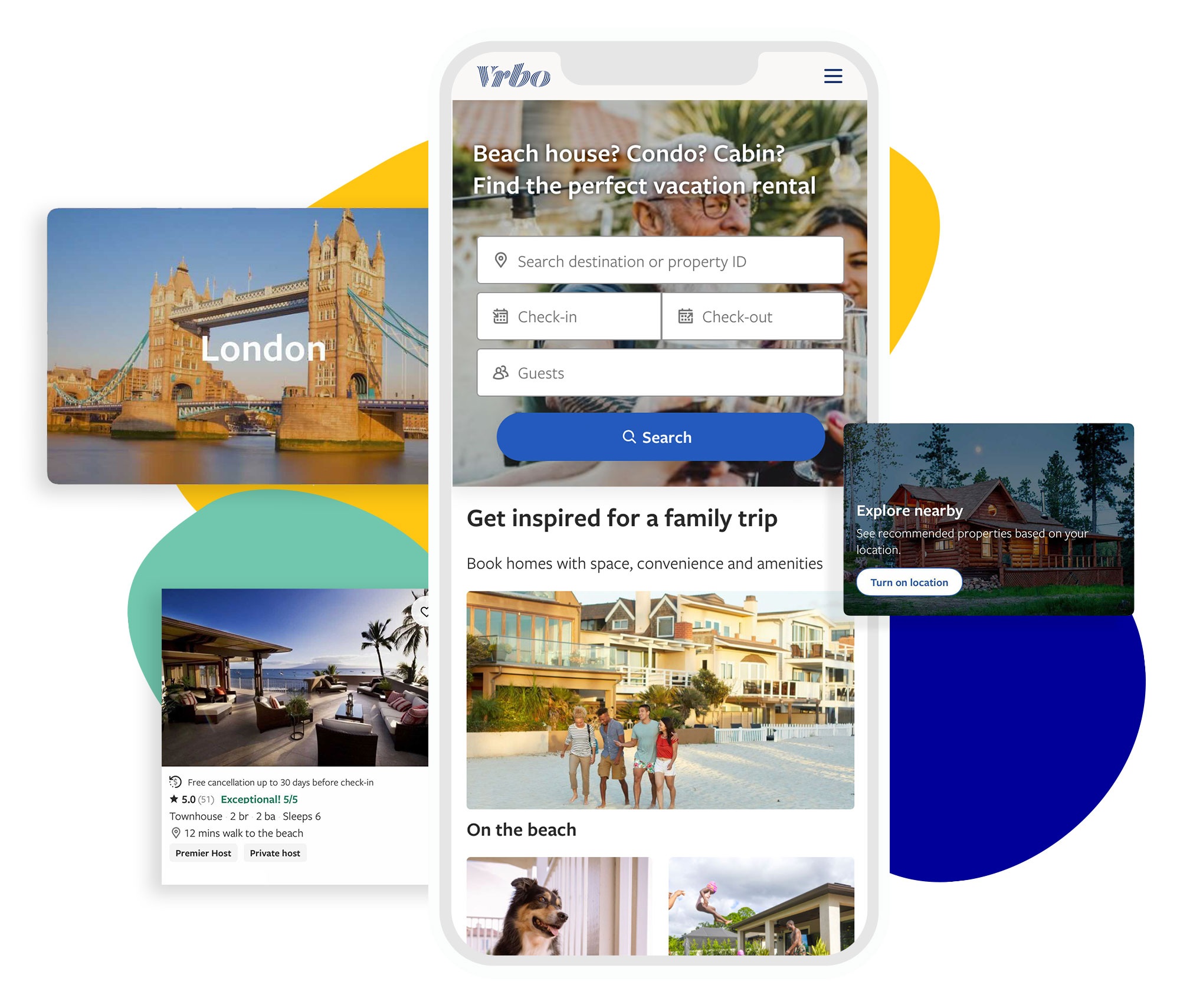This promotional image for Vrbo showcases various attractive vacation rental options and features. At the center of the image, there's a white and gray-toned cell phone design. In the upper left-hand corner, the Vrbo logo is prominently displayed. Below the logo, in white font, the text highlights different types of vacation rentals available: "Beach House, Condo, Cabin."

A search bar is prominently displayed, inviting users to "Find the Perfect Vacation Rental" by searching using a destination or property ID, along with options to input check-in and check-out dates and the number of guests. A prominent "Search" button emphasizes user interaction.

Below this section, the text encourages potential customers with a message: "Get inspired for a family trip. Book homes with space, convenience, and amenities." A picturesque image of four people walking along a beach, flanked by beautiful beachside homes, complements this message.

On the right side of the image, a nighttime shot of a cozy log cabin nestled among tall trees is paired with text encouraging users to "Explore Nearby." It suggests discovering recommended properties based on their location and prompts users to turn on their location settings for more personalized results.

In the upper left section, an image of a large bridge is captioned with "London," indicating international rental options. At the bottom left, an inviting outdoor beach setting with palm trees is further detailed with enticing information about a specific rental property: "Free cancellation up to 30 days before check-in. Townhouse, two bedroom, two bath, sleeps six. 12-minute walk to the beach. Premier host, private host, with a five-star review."

The overall aesthetic of the advertisement is designed to entice potential renters with a mix of beautiful imagery, highlighted features, and user-friendly search functionalities.